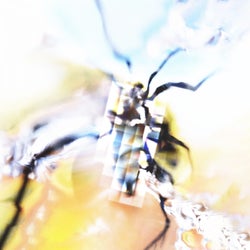The image depicts a highly zoomed-in and blurred object that appears insect-like, possibly a bug, overlaid with a grid pattern of small, colorful cubes, making it look distorted or pixelated. The central figure, which resembles a bug, has black lines extending from it, reminiscent of legs or antennae. The object has sections that feature an orange-yellow gradient at the bottom, transitioning to a pinkish salmon color, and finally into a light blue background in the upper portion, which is streaked with darker blue and white veins. The overall effect is reminiscent of an AI-generated image or an abstract, kaleidoscopic representation, presenting an eclectic mix of colors including yellow, light pink, purple, and beige, overlaid with a textured grid.